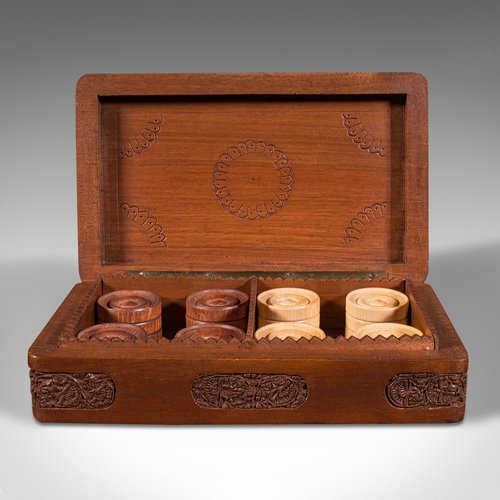The photograph depicts an antique wooden box, intricately carved with detailed floral motifs, both on the front and the interior of the lid. The open box reveals two compartments, each divided by a wooden slat. Inside these compartments are stacked circular wooden pieces, possibly checkers or markers. The left compartment holds darker brown pieces, while the right compartment contains lighter, almost pale, cream-colored pieces. Each stack consists of around three to four pieces, arranged in four stacks per side. The entire scene is set against a neutral white and gray background.